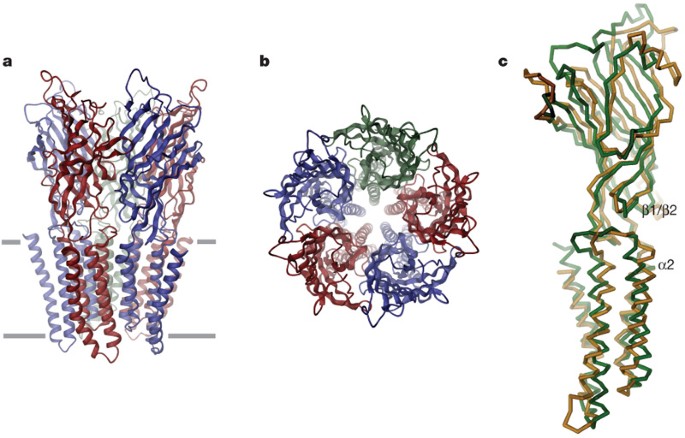The image features a scientifically detailed illustration of open-state proton-activated pentameric ligand-gated ion channels, segmented into three labeled parts: A, B, and C, from left to right, set against a white background. In part A, vibrant ribbons, predominantly red and blue, intertwine vertically resembling curlicue spirals or towers. Part B presents a circular arrangement of the same ribbon-like structures in red, blue, and green, forming an intricate star-like or octagonal pattern. Part C depicts more dispersed and thin ribbons in shades of green, brown, and amber, annotated with B1/B2 and A2 symbols. This colorful yet complex visualization captures the dynamic and structural diversity of the protein channels, highlighted by the different visual arrangements and the detailed labeling.